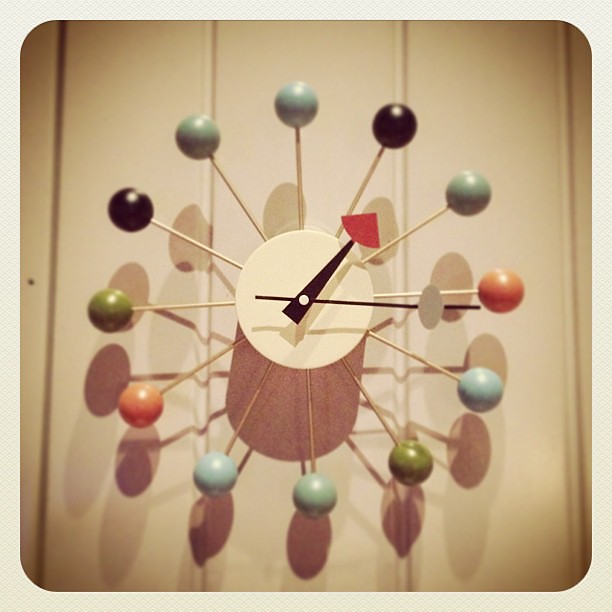This detailed photograph depicts a mid-century modern sculptural clock, characteristic of the 1950s or 60s vintage style. The clock features an inner cream-colored circular face with a sleek design. Radiating from this center are twelve slender, light tan or yellowish wooden dowels, each extending outward to represent the hours of the day. At the end of each dowel is a colored ball, painted in hues of blue, green, orange, or black, adding a playful yet sophisticated touch to the abstract design.

The clock's hands are geometric and minimalist, with the hour hand being a black triangle ending in a red arrow, pointing towards the top right. The minute hand is a skinny black stick, extending just past the 3 o'clock position. The entire piece is mounted on a backdrop of white wall paneling, featuring three prominent vertical wooden planks, giving the composition a clean and modern aesthetic. This photograph captures the essence of mid-century interior design, with muted tones and geometric shapes that evoke a sense of timelessness.